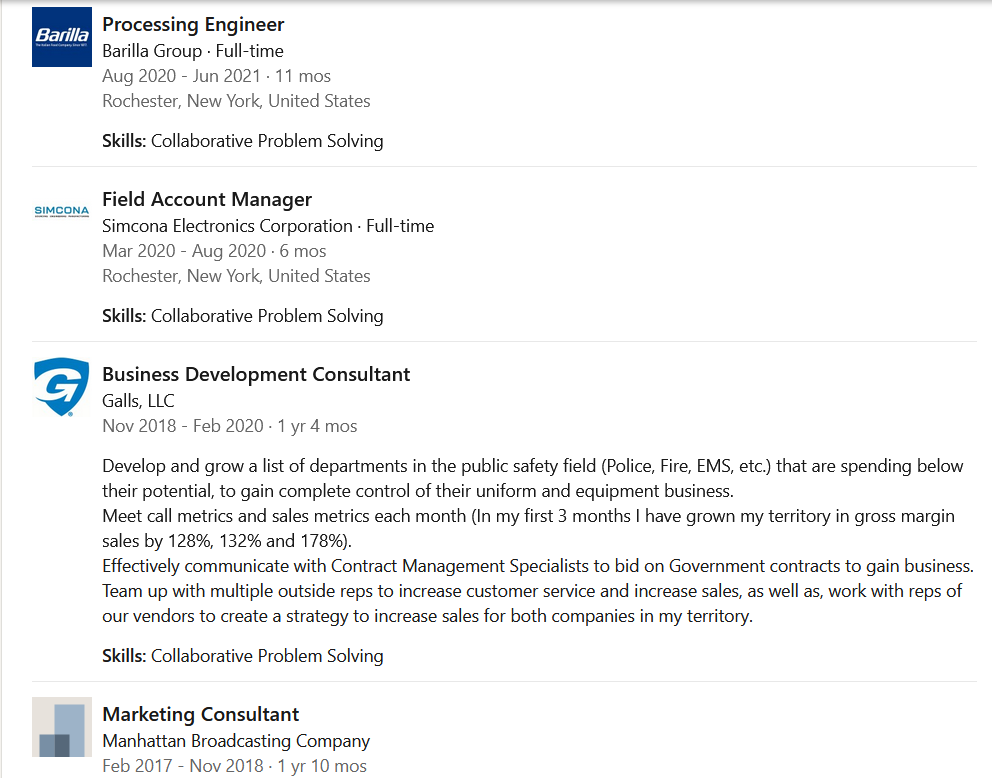The image features a white background with a light blue outline along the top and left edges. At the top, there is a blue box with the text "Borilla" inside, accompanied by "Processing Engineer, Borilla Group, full-time, August 2020 to July 2021, 11 months, Rochester, New York, United States." It also highlights the skill "Collaborative Problem Solving."

Below this, a small separator line precedes details on another role: "Field Account Manager, Simcona Electrics Corporation, full-time, March 2020 through August 2020, 6 months, Rochester, New York, United States," also emphasizing the skill "Collaborative Problem Solving."

Next, a blue shield icon with a "G" inside it denotes a third position: "Business Development Consultant, LLC, November 2018 through February 2020, 1 year, 4 months." The description elaborates on the responsibilities, including developing and growing a list of public safety departments that are under-spending, meeting monthly call and sales metrics, and achieving significant territory growth in gross margin sales by up to 178%. It also highlights the ability to effectively communicate with contact management specialists to secure government contracts and collaborate with multiple teams to boost sales and customer service. The skill listed is "Collaborative Problem Solving."

The last section features a light blue box containing three other boxes in varying shades of blue, describing the position "Business Development Consultant, Manhattan Broadcasting Company, February 2017 through November 2018, 1 year, 10 months."